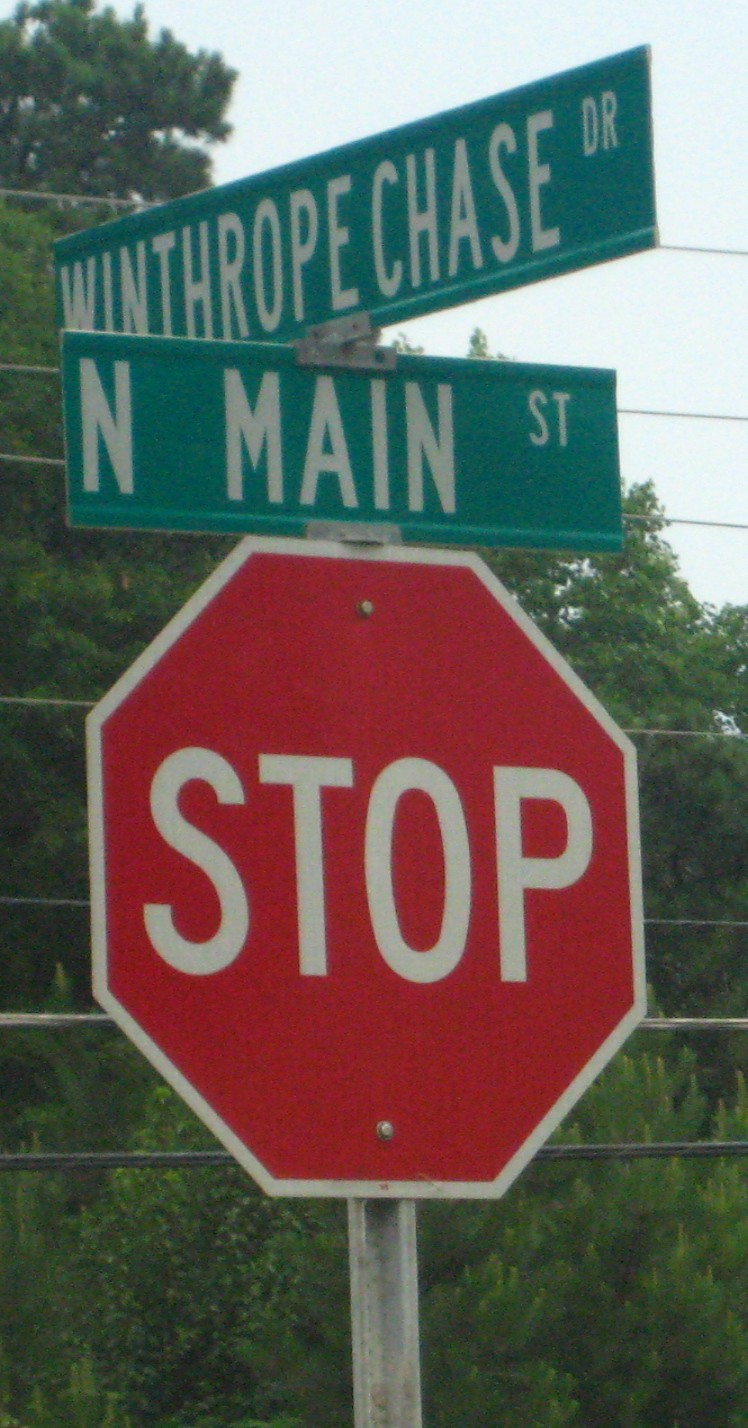This vivid photograph captures a classic red and white octagonal stop sign, prominently displayed against a backdrop of lush greenery. The sign is emblazoned with the word "STOP" in bold white letters, clearly visible at its center. It is securely fastened with a shiny silver screw to a sturdy metal post, which extends from the sign's base to the bottom of the image. Behind the stop sign, six horizontal, silver-colored lines add a striking visual contrast. Topping the stop sign are two green rectangular street signs; the upper one reads "Winthrop Chase Drive," while the one below it indicates "North Main Street." The scene is framed by vibrant green trees and a glimpse of sky in the top right corner, enhancing the overall composition with a touch of nature.